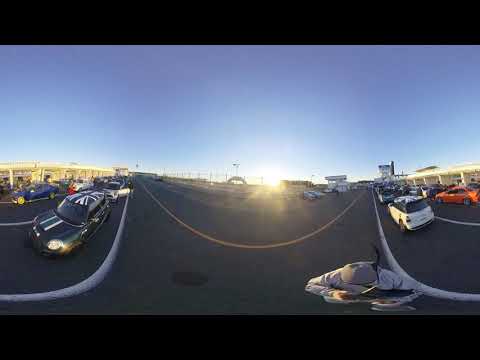The image depicts a distorted, fisheye view of a roadway, as if seen through a peephole. The foreground shows a human figure wearing a gray beanie and a white sweatshirt or hoodie, standing near the middle of the road. The road features distinct traffic markings, with a curved yellow center line and six white solid lines, although only five are clearly visible.

On the left side of the image, a black car with a British flag painted on its roof is parked, its headlights on. Behind it, another car with a silver exterior has its door open, with a person in a black shirt and white pants standing beside it. Additionally, a blue car is visible near these, with several people standing behind it.

Toward the right, a white car with two wheels showing is parked next to an orange car. Several other cars, both silver and blue, are scattered around. In the background, the sun is setting, illuminating the clear blue sky with a warm light. Two white structures, presumably buildings, flank either side of the image.

In the bottom right corner, another person can be seen, also dressed in a beanie and hoodie. The overall composition suggests a bustling scene, possibly a parking lot, with various people and vehicles caught in a momentary, distorted perspective.